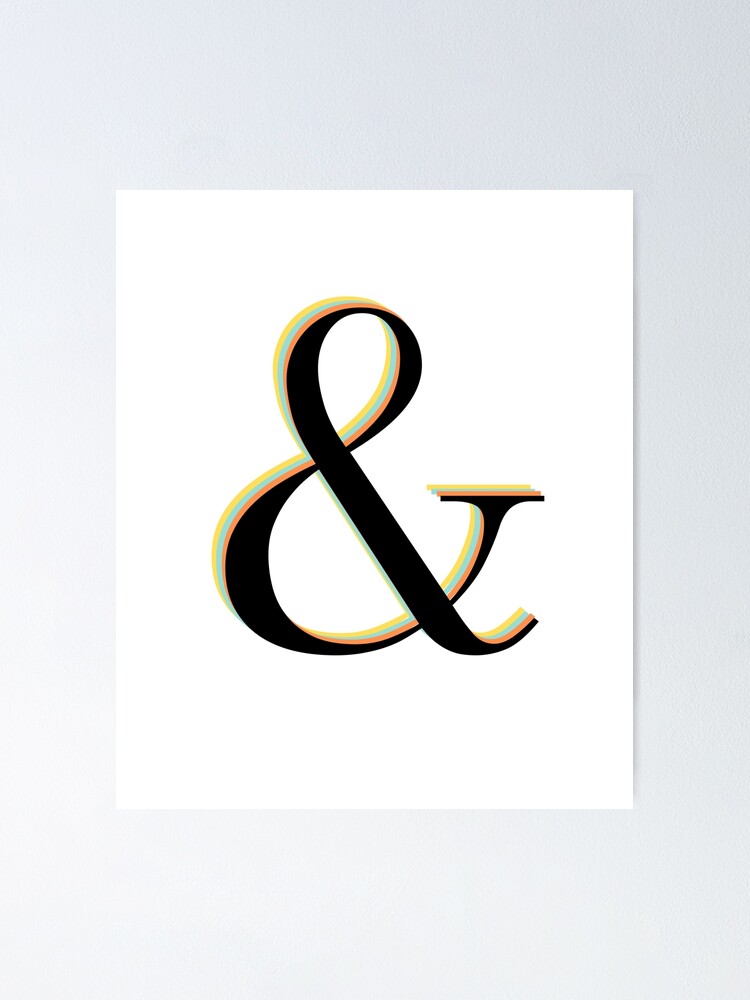The image depicts a photograph of another photograph, both in a rectangular format. The outer photograph is approximately six inches tall by four inches wide and features a light gray border that fades to white towards the bottom. Positioned centrally within this border is a smaller, pure white rectangle, reminiscent of a sheet of paper, which measures about two inches wide and three inches high. Centered in this smaller rectangle is a prominent black ampersand symbol. This black ampersand is accentuated by a multi-colored shadow outline that gives the symbol depth and dimensionality. The shadow outline consists of three colors arranged in order: a peachy orange closest to the ampersand, followed by light blue, and then light yellow gold, creating a striking visual effect against the white background. There are no additional borders, symbols, watermarks, or signatures present in the image.